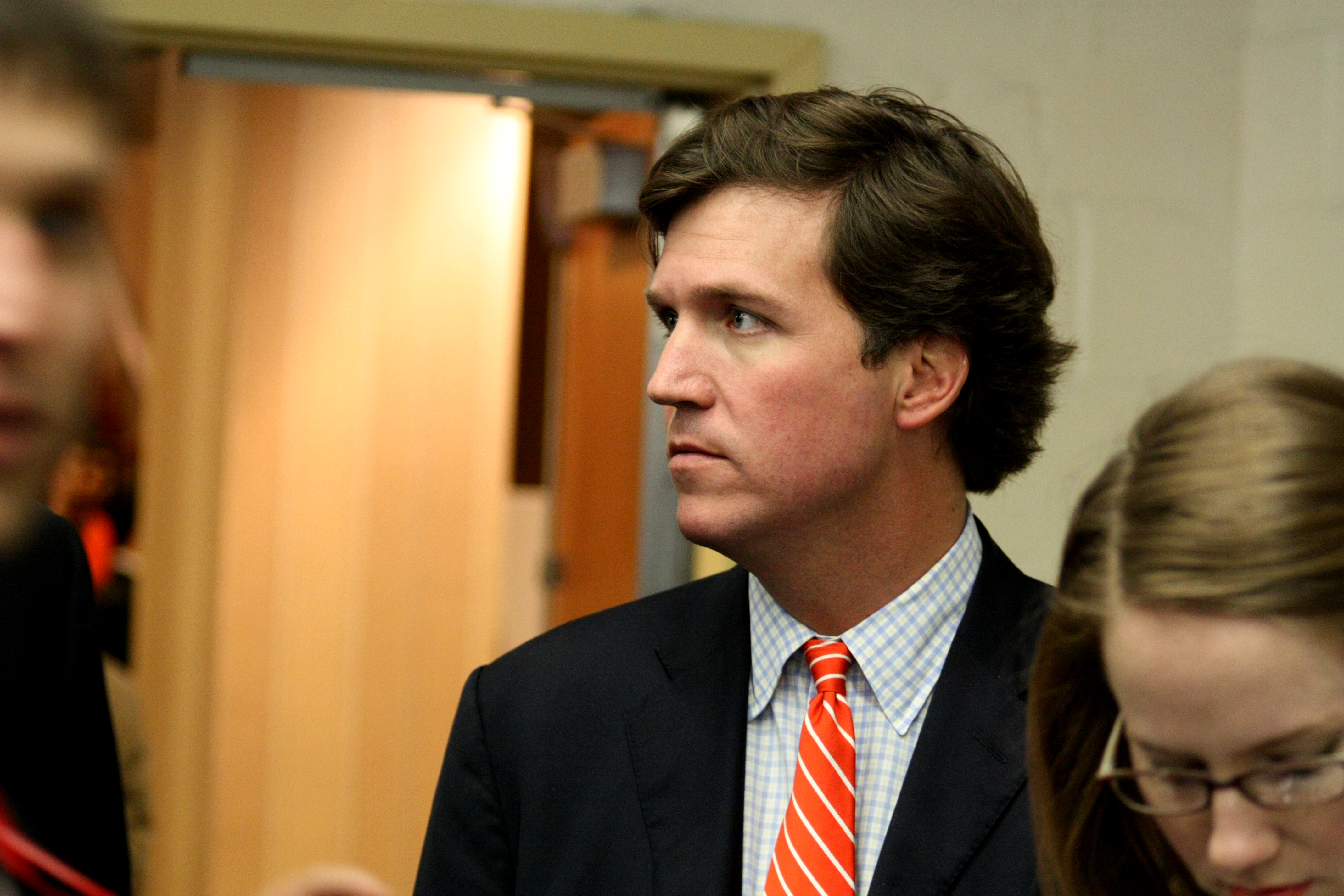The image features a profile view of a man with wavy, short brown hair positioned near the right side of the frame. He is looking to the left with an intense expression on his face. The man is dressed in a blue and white checkered button-down shirt paired with a red and white striped tie and a dark jacket. Standing next to him, a woman with long, straight blonde hair and glasses is looking down. She appears near the lower right corner of the image. The background includes a light-colored wall and a closet door or wooden door. Additionally, on the left side of the image, there is a blurred section displaying part of another man's face and upper body.